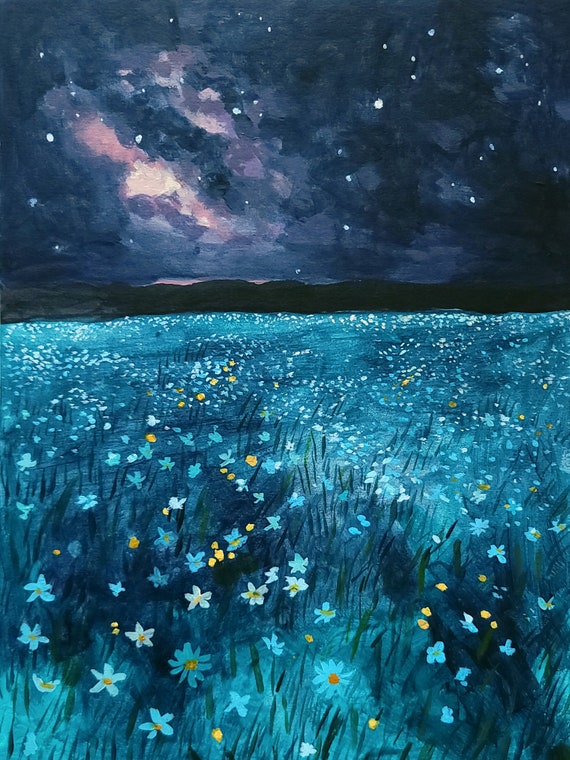This detailed watercolor painting captures an enchanting nighttime scene set in a vibrant, flower-filled field with low, distant mountains beneath a star-studded sky. The foreground bursts with a variety of flowers, including blue daisies and those with white petals and yellow-orange centers, shaped like crosses, intermingled with tall green stalks of grass, though the field itself exudes an overall blue hue with scattered green and white speckles. The painting's lower half focuses on this rich floral tapestry, while the midground introduces a series of dark, rolling hills. The blue and orange sky above, tinged with hints of purple, hosts a multitude of white stars peeking through cloud wisps, suggesting the gentle glow of the moon. The vertical rectangular composition has no text or artist signature, emphasizing the scene's captivating beauty and serene nocturnal ambiance.